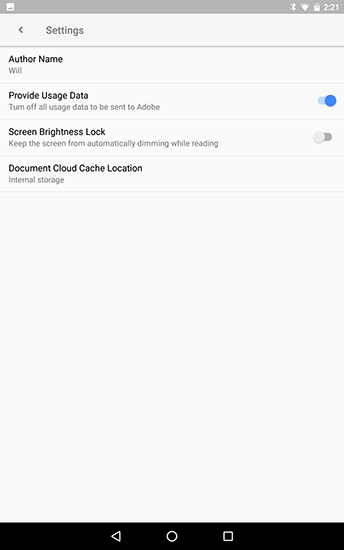A small, black and white screenshot of a mobile device displays various settings and options against a gray background. At the top, a gray bar spans across the screen, showing "221" with an indicator of "good strength" and a "Settings" label accompanied by a left-pointing arrow. Below this, a thin gray bar marks an area with additional text: "author's name" in smaller font, followed by several options related to data and screen management.

Highlighted settings include:

1. "Provide usage data": A toggle switch located beside this option is illuminated in blue, indicating it is currently active. The accompanying description reads, "Turn off all usage data to be sent to Adobe."
2. "Screen brightness lock": An option to "Keep the screen from automatically dimming while working" which is turned off.
3. "Document & cloud cache location": Displays "internal storage" as the selected option.

The lower portion of the image shows no text or images, filled only with a plain gray background. At the bottom of the screen, the usual navigation icons typical on Android devices are visible: a home button (circle in the middle), a back arrow (pointing to the left), and a recent apps box (outlined in white) all set against a dark black strip.

The image lacks any additional information, such as a company name or specific context for the settings shown, leaving the purpose of these options unclear.